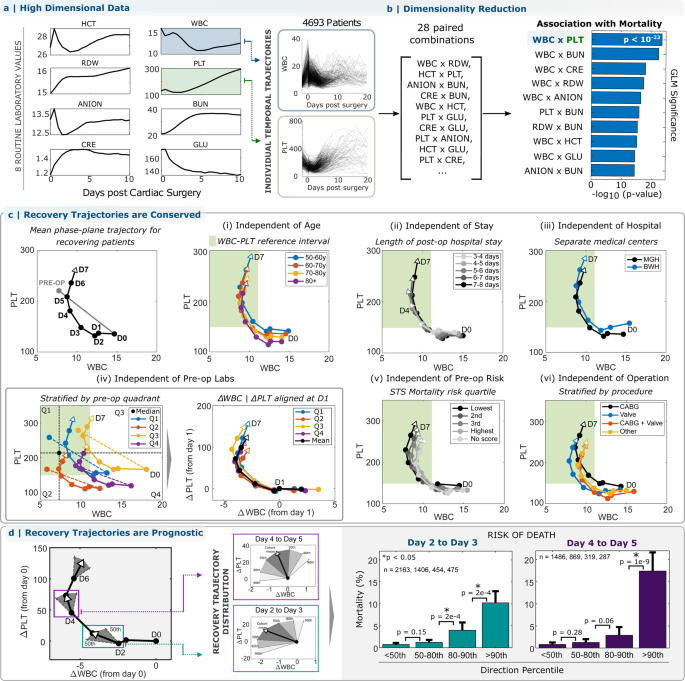The image displays a complex set of scientific diagrams organized into four distinct sections labeled A, B, C, and D, each containing various charts and graphs. Section A, titled "High Dimensional Data," features line charts and focuses on data involving routine laboratory values, dimensionality reduction, and associations with patient mortality. Section B, named "Dimensionality Reduction," includes an array of grid charts and bar charts, and is noted to include 28 paired combinations. Section C, titled "Recovery Trajectories are Conserved," presents segmented line graphs depicting individual patient data such as age, length of stay, and hospital information. Section D, labeled "Recovery Trajectories are Prognostic," contains additional charts and detailed descriptions related to patient recovery outcomes. The entire image sits on a white backdrop with very limited use of color, emphasizing its scientific and analytical nature.